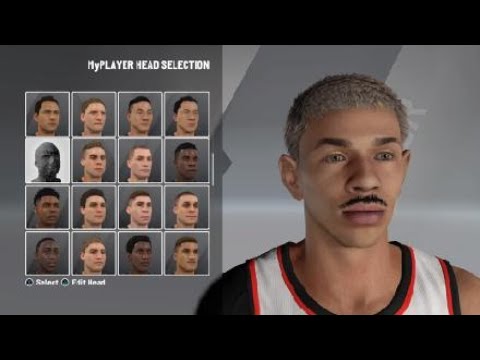Screenshot of an NBA 2K24 player optimization screen, featuring a detailed player selection interface. The top of the screen has an edited-out section where the player's name would typically be displayed. To the right, in bold white capital letters, it reads "PLAYER HEAD SELECTION." Below this, there are four rows of four different head types each. The first head on the second row is selected, indicated by a grayed-out box. At the bottom of these rows, options to select or edit the head are visible.

On the right side of the screen, the player's head and shoulders are shown in focus. The player sports very short, almost completely shaved blonde hair and a black mustache. He is dressed in a white jersey with black and red accents tracing the neckline and sleeves. The screenshot is framed with black borders at the top and bottom, adding a polished look to the captured image.